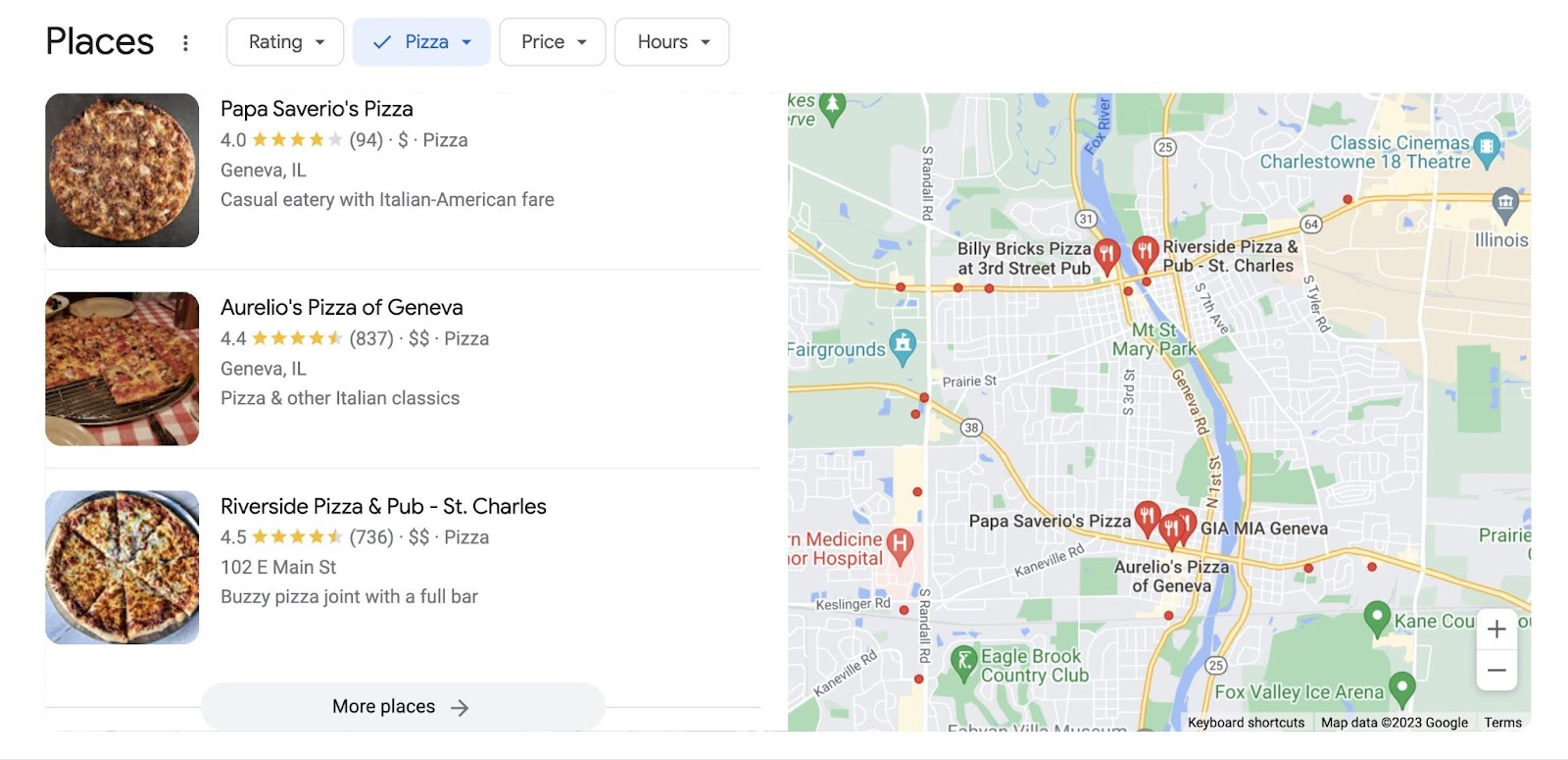The image displayed is a Google search result page showcasing various pizza eateries in Geneva, Illinois. The webpage includes a section labeled 'Places' with a filter box containing options such as ratings, price, and hours. The 'pizza' filter is highlighted in blue with a checkmark beside it. 

Below this, there are listings for different pizza establishments: 

1. **Papa Saverio's Pizza** 
   - Rating: 4 out of 5 stars
   - Reviews: 94
   - Description: A casual eatery serving Italian-American fare.

2. **Aurelio's Pizza of Geneva**
   - Rating: 4.4 out of 5 stars
   - Reviews: 837
   - Location: Geneva, Illinois

3. **Riverside Pizza and Subs**
   - Rating: 4.5 out of 5 stars
   - Reviews: 736
   - Location: 102 East Main Street, St. Charles
   - Description: A buzzy pizza joint with a full bar.

On the right side of the search results, there is a Google Maps image with location pins marking the different pizza places, providing a visual representation of their locations.